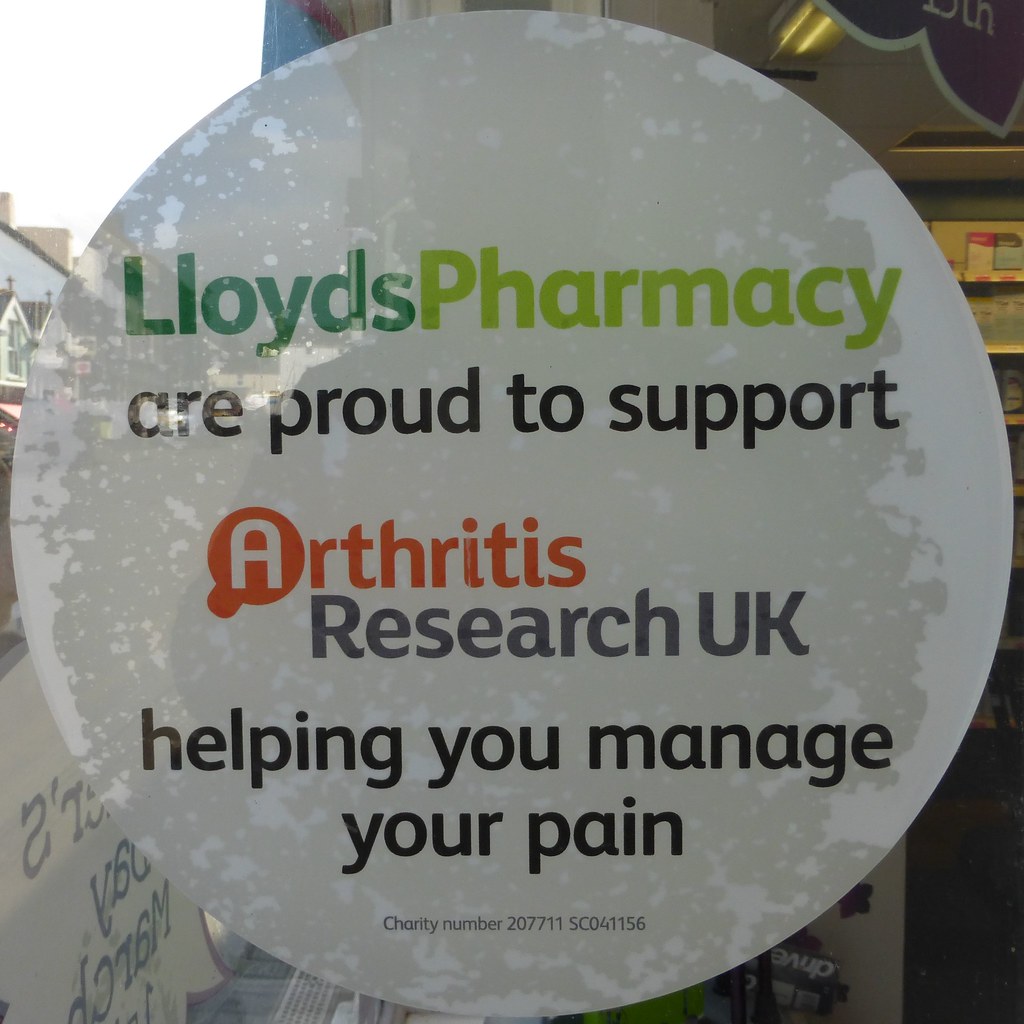The image shows a large, circular sticker with a marbleized white and gray background, which takes up most of the frame. The sticker prominently displays the text: "Lloyd's Pharmacy are proud to support Arthritis Research UK, helping you manage your pain," followed by the charity number "207711 SC041156." The text is multi-colored, featuring green, red, black, and gray. The sticker appears to be situated on the inside of a store window, likely a pharmacy, indicated by the glare on the glass. Surrounding the sticker, additional stores and businesses are visible in the background.